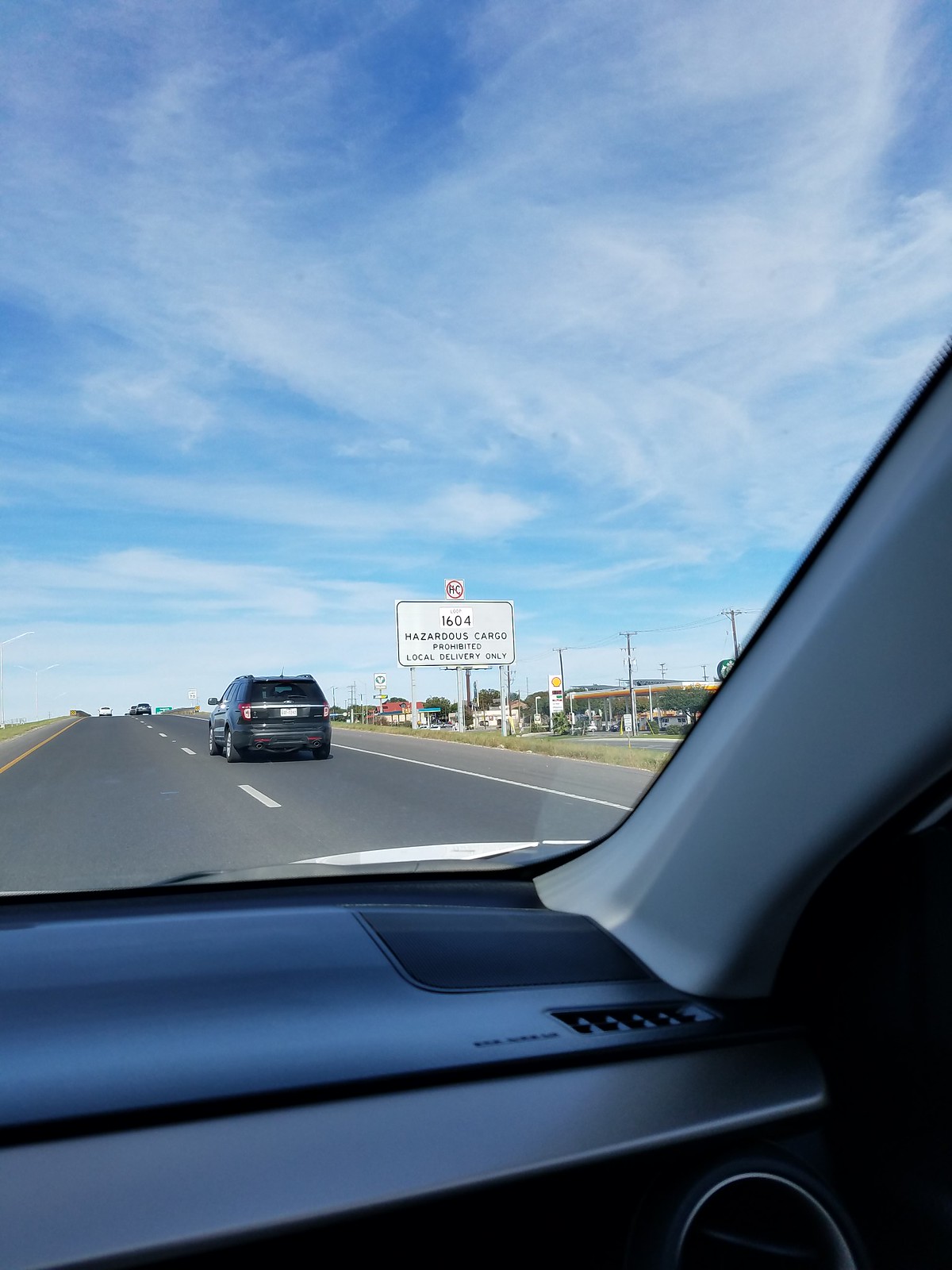A breathtaking view from the passenger side of a car traveling on a two-lane highway on a clear day. The extremely blue sky is adorned with sweeping white clouds, creating a picturesque backdrop. In the lower right-hand corner of the windshield, a large white road sign mounted on a steel rod stands out. The sign is outlined and bordered in black with bold black writing, topped with a small red attention-getter to ensure visibility. A strip of grass lines both sides of the road, adding a touch of greenery to the scene.